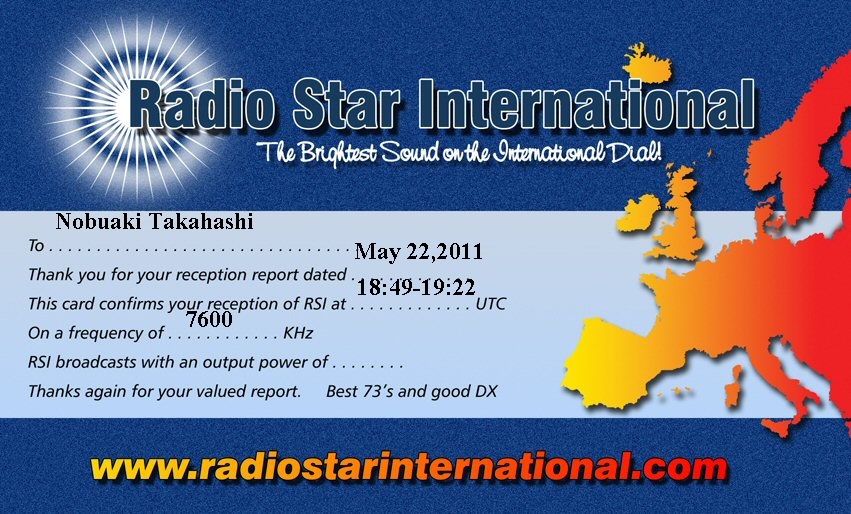The advertisement is a horizontal rectangle with a predominantly dark blue background that lightens towards the center. At the top left corner, there's a glowing white spot with radiating lines, creating a visual focal point. Encircled by an alternating pattern of dark and light blue rings, this spot fades seamlessly into the blue background.

Across the top, the words "Radio Star International" appear in dark teal with a white outline. Beneath that, the tagline "The brightest sound on the international dial" is written in white cursive. Beneath the tagline, a large light blue banner contains black text stating "Nobuaki Takahashi to May 22, 2011. Thank you for your reception report dated 18:49 to 19:22 UTC. This card confirms your reception of RSI at a frequency of 7600 kHz. RSI broadcast with a power output of [blank]. Thanks again for your valued report. Best 73s and good DX."

On the right side of the advertisement, there's a depiction of Europe, highlighting the broadcast's reach from Spain through the UK and into Ireland. The bottom of the image features the website "www.radiostarinternational.com."